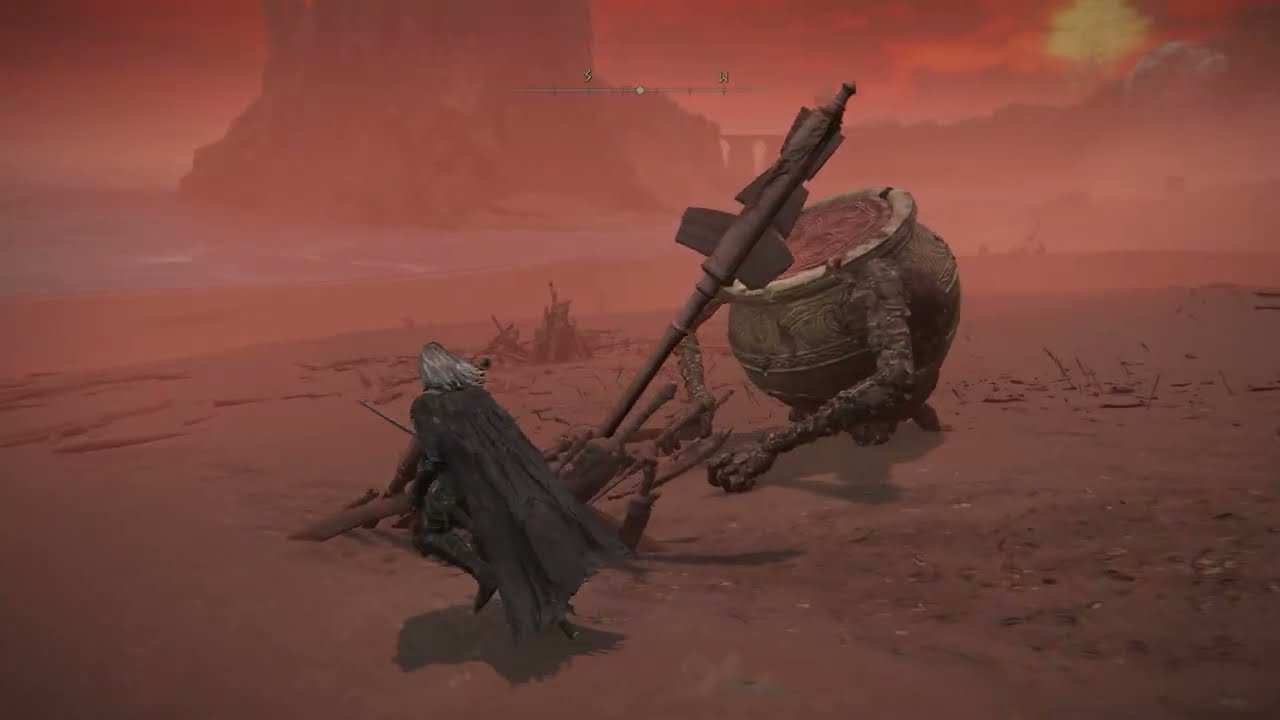The image is a wide, rectangular, computer-generated illustration in a fantasy world, predominantly colored in shades of red, brown, orange, and gray. The bottom two-thirds of the scene features a dark, barren, reddish-brown terrain scattered with occasional piles of sticks and stumps. Centered from the left, a character resembling the Witcher—distinguished by his long, flowing silver hair and tattered black cape—runs across the desolate landscape, heading towards the top left. Chasing him from the right, a spherical, robot-like entity with dark gray metallic arms is holding a weapon. Behind them, a tumultuous red and gray body of water reflects the ominous sky, which is ablaze with blood-red clouds and a distant yellow sun. Far in the background, between two large mountain ranges, the silhouette of a Grecian-columned building emerges through the mist. The overall tone of the image is bleak and menacing, weaving elements of illustrative surrealism and dark fantasy, suggestive of an otherworldly video game scene set in a post-apocalyptic desert.